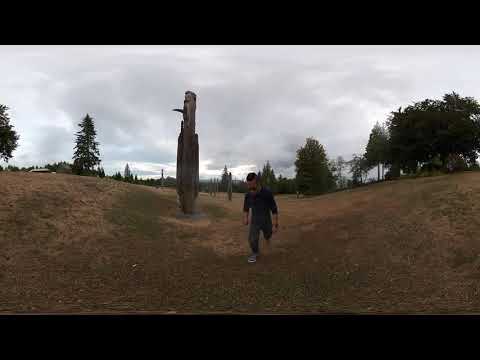This rectangular photograph, framed with solid black bars at the top and bottom, depicts a gloomy, overcast scene with a sky blanketed in gray clouds, creating a pre-storm atmosphere. In the center of the image, there is a man, seemingly Caucasian with dark hair, wearing dark-colored clothing, including a long-sleeved black shirt, black pants, and gray sneakers. His posture suggests he is running towards the viewer, his right foot planted firmly with his back leg extended behind him, giving the impression of movement down a hill through a partially hilly landscape. The terrain underfoot is a mix of brown dirt and sparse green grass, indicative of early spring or winter. To his right and slightly behind him stands a tall, narrow wooden totem, twice his height, possibly carved to resemble a human form with distinguishable facial features like a protruding nose. A few scattered trees dot the barren landscape in the background, adding to the desolate feel of the scene.